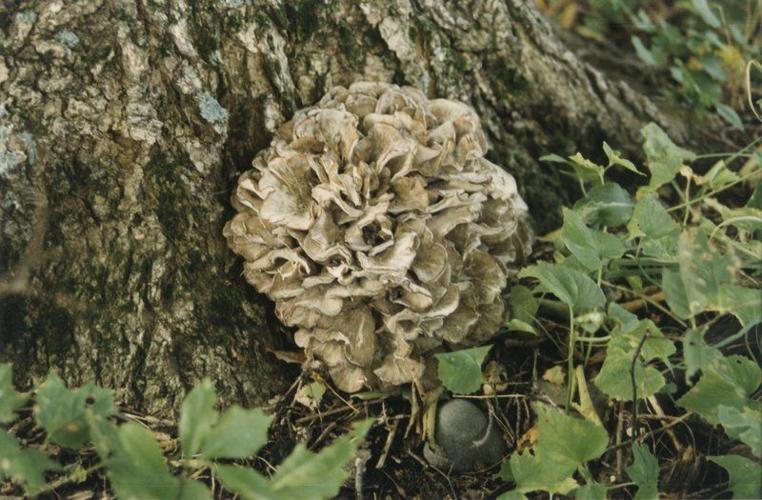A close-up photograph captures the base of a rough-barked tree trunk partly surrounded by green leaves and dirt. Dominating the center of the image is a large, whitish-gray mass resembling either a hydrangea flower or possibly a dense cluster of small mushrooms fused together, indicating some form of fungus. This intriguing growth rests directly at the base of the tree trunk, with varied green foliage, both dark and light, encircling it. To the side, a notable gray rock lies prominently near the bottom edge of the frame. The stems of the surrounding plants are intermingled with the leaves, some of which are visible towards the upper right. The scene is an intimate glimpse at the ground-level life of this natural habitat, highlighting the close interplay between the tree, the enigmatic fungal growth, and the lush greenery.